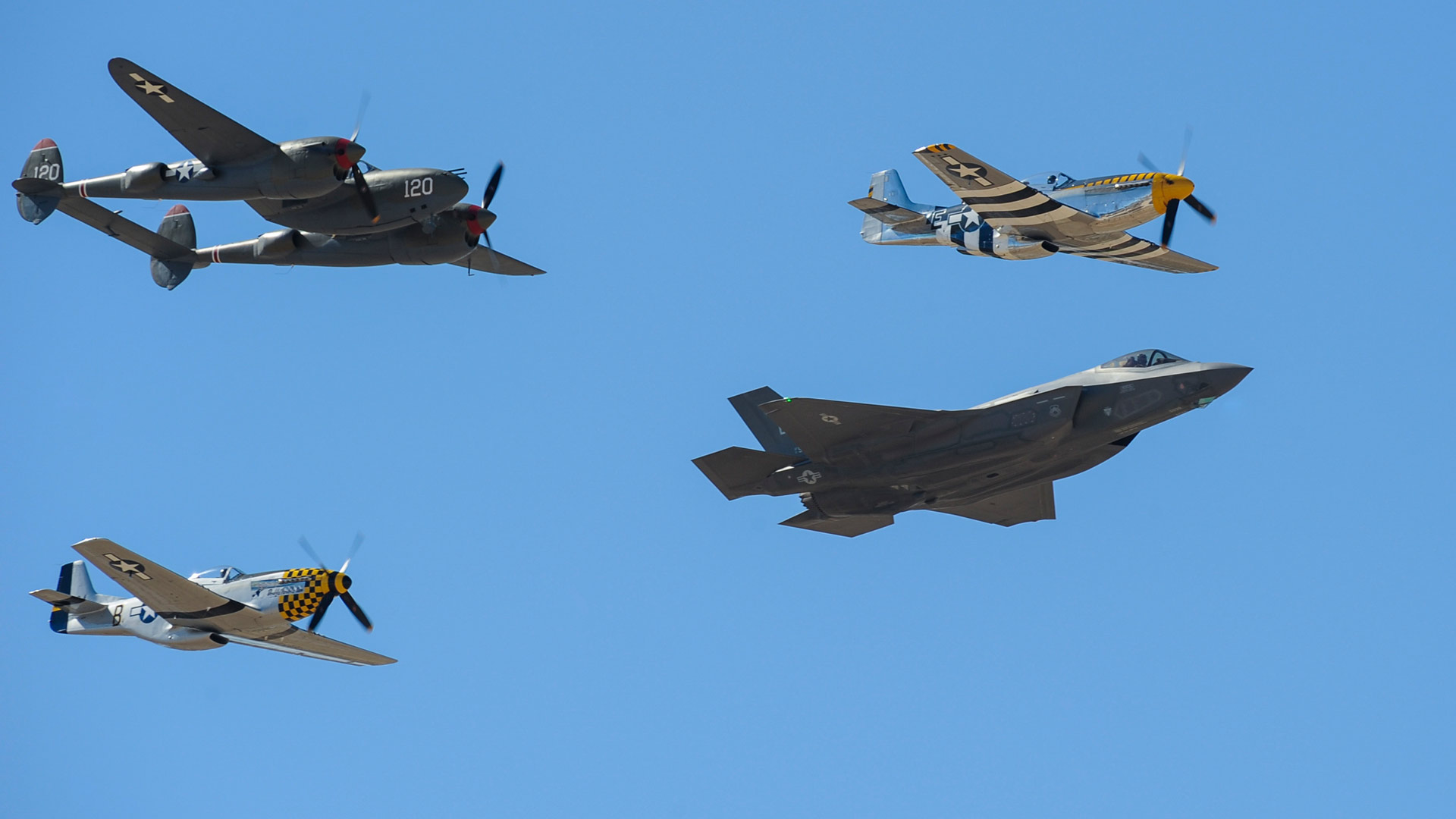In this striking image captured against a vibrant, cloudless blue sky, four aircraft are flying in close formation, presumably at an airshow. On the upper left is a vintage P-38 Lightning, distinguishable by its dark gray color, twin booms, horizontal stabilizer, and two front propellers. This aircraft bears the number 120 and features the white star-and-stripe insignia characteristic of American livery. Shining brightly in a metallic silver, the upper right and lower left corners are occupied by two P-51 Mustangs. These planes sport yellow nose tips, checkered patterns, and similar star-and-stripe symbols beneath the wings and on their sides. Lastly, positioned more toward the center but to the lower right in the grouping, is a modern F-35 jet. This sleek, triangular-shaped aircraft is entirely gray and lacks propellers, embracing the streamlined design of contemporary fighter jets. The tight formation hints at a dynamic and choreographed flight display, celebrating the craftsmanship and evolution of military aviation.